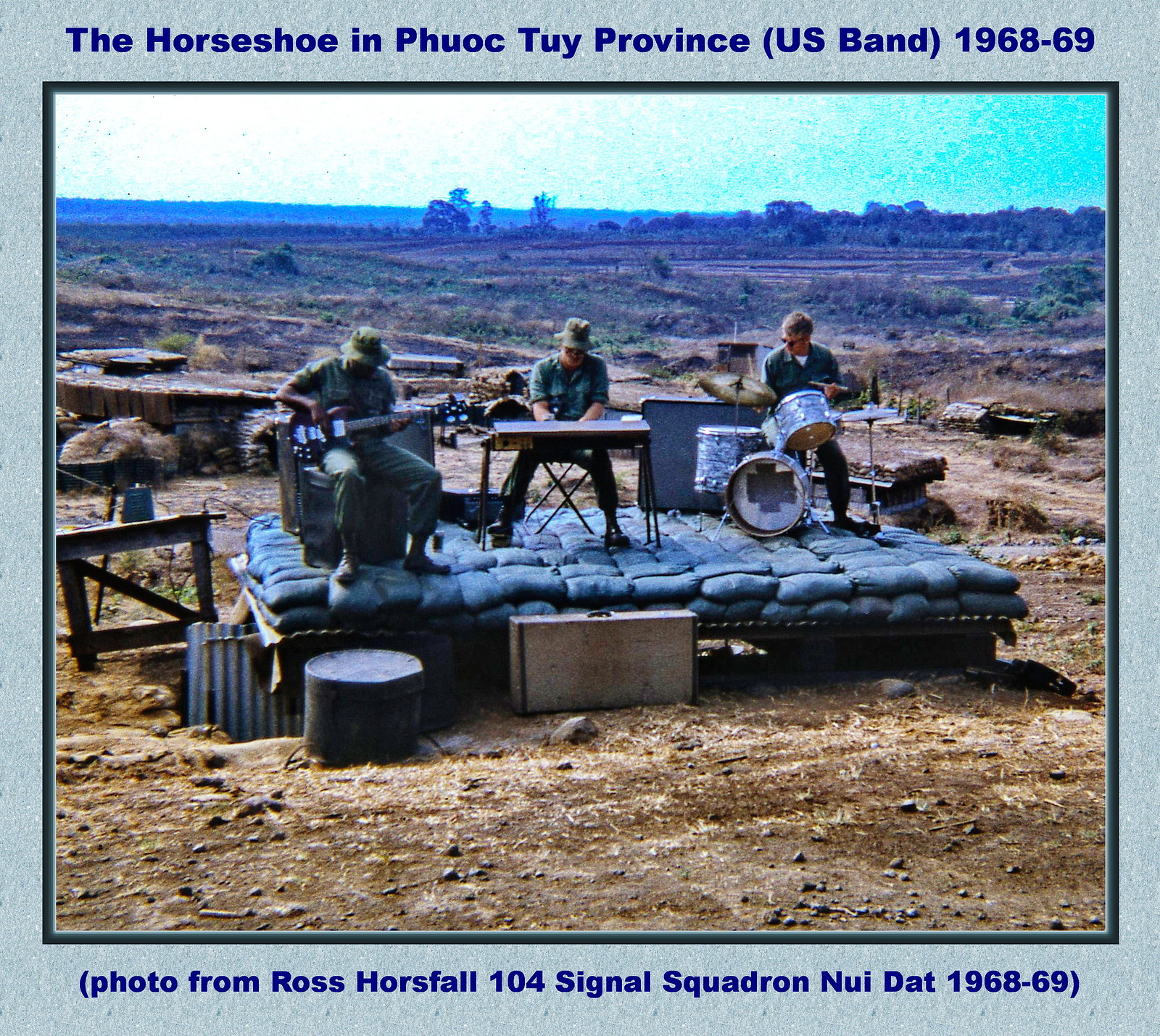The image shows a makeshift stage in a desert-like terrain, with sparse vegetation, lots of dirt, and a few shrubs, likely in Vietnam during the years 1968-69. The stage, made of stacked cloth sandbags or bedding, holds three seated musicians in army outfits: a guitarist on the left, a keyboard player in the center, and a drummer with silver drums on the right. In front of the stage is a speaker, and to the left, a few rocks are visible. The light blue background of the picture features blue text at the top, reading “The Horseshoe in Phuoc Tuy Province, U.S. Band, 1968-69,” and at the bottom, it states “Photo from Ross Horsefall, 104 Signal Squadron, Nui Dat, 1968-69.”